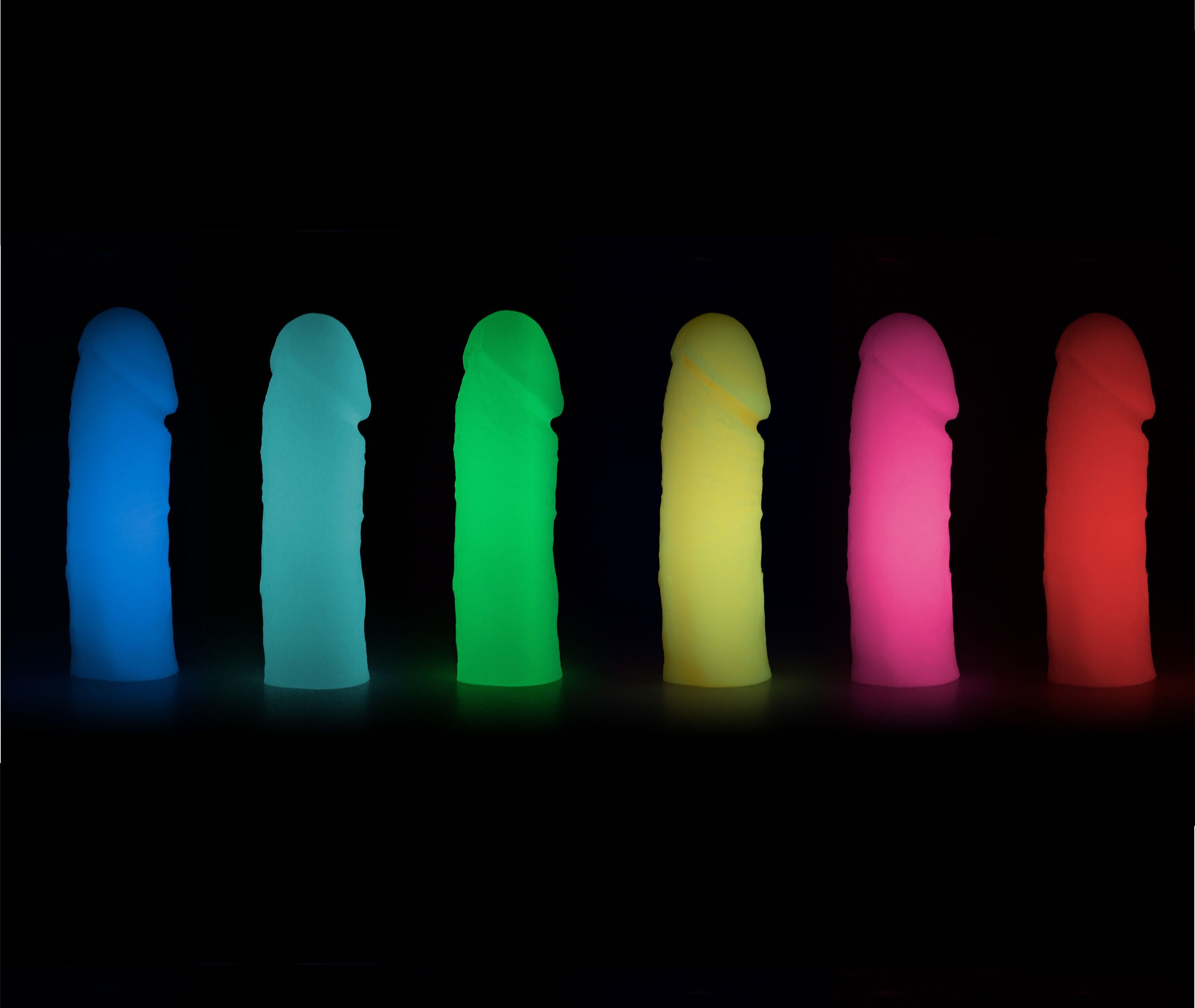This photograph features six glow-in-the-dark dildos arranged in a neat line against a completely black background. The dildos are positioned vertically on what appears to be a black platform, with each one spaced approximately an inch apart. From left to right, the colors of the dildos transition sequentially through dark blue, light blue, neon green, yellow, pink, and red. Each dildo is identical in shape and size, with a uniform width along their entire length and flat ends, suggesting they lack a traditional base. The vibrant colors stand out starkly against the dark backdrop and cast slight colored shadows on the surface below them, emphasizing their luminescent, neon quality.